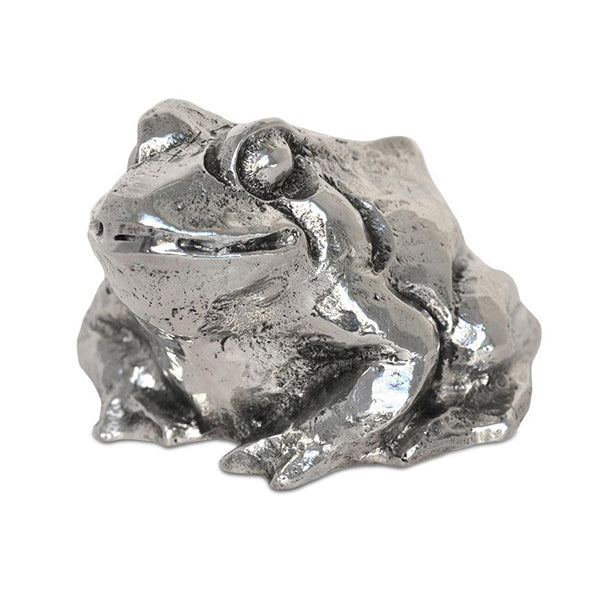The image showcases a decorative silver frog sculpture centered against a plain white background. This shiny, possibly metal or glass object, features a three-quarter profile view, facing slightly to the left. The frog has large, silver eyes positioned on top of its head, gazing outward. Its characteristic broad, subtly smiling mouth displays a distinctive separation between the top and bottom lips. The sculpture is detailed with a series of smooth and rough patches, as well as dimples scattered throughout its surface. The frog’s front legs and hands are visible, with a slight hunch on its back. While minimal in detail, the shape and form unmistakably depict a frog, capturing a charming yet abstract essence.